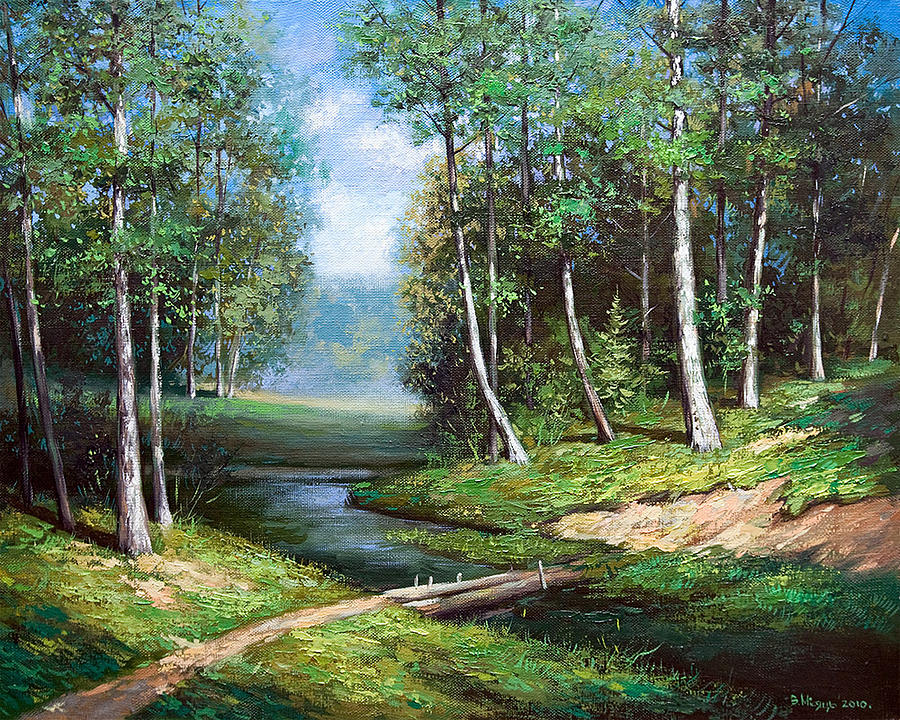This painting captures a serene outdoor woodland scene, likely in spring or summer, with lush greenery throughout. The foreground features a gentle hillside on the right, covered in patches of light and dark green grass. There are four slender trees with light gray, patchy trunks that gradually give way to branches higher up. To the left of the viewer, the hillside slopes down toward a tranquil creek or little waterway that winds through the landscape.

A light and dark brown log bridges the creek, connecting the grassy areas on both sides. The grassy banks on either side of the creek are dotted with numerous trees, their slender, dull brown trunks also displaying speckled white patches. The background reveals a cluster of additional trees, enhancing the dense woodland ambiance.

Above this peaceful scene, a bright blue sky stretches across the horizon, adorned with fluffy white clouds, some tinged with shades of gray. There is also a hint of fog near the ground in the distance, adding a touch of mystique to the calm and inviting landscape.